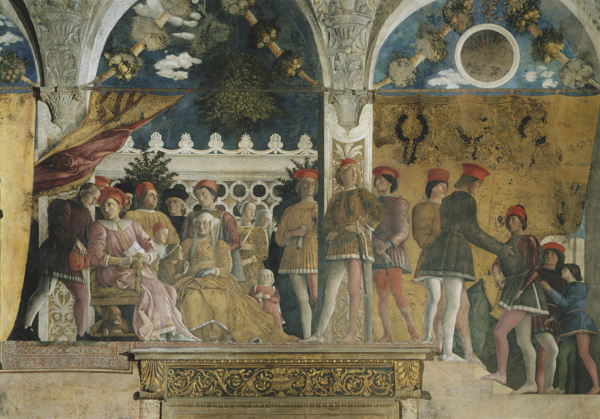The image depicts an ancient painting featuring a grand, ornate setting that resembles a royal palace, characterized by intricate, curved arches and cloud-covered blue skies. Prominent in the painting are concrete pillars that stretch around the scene, supporting the artistically rendered architecture. The ornate furniture and detailed surroundings suggest a representation of a royal or religious gathering. The attendees, a diverse group comprising men, women, and children, are all adorned in robes and flat red hats, which unify their appearance. Their attire includes long gowns in hues of yellow, pink, and brown, with some women notably wearing leggings. The scene is filled with various activities—some individuals are seated, a few are walking, and there's a notable figure in a dark brown shirt and skirt wearing tights, gazing at a woman in a pink robe beside him. The backdrop also includes lush hanging plants and sections with white fences decorated with circular patterns. A light yellowish-brown backdrop with potential map-like designs and various rods descending from the arches add to the elaborate detail of the artwork.